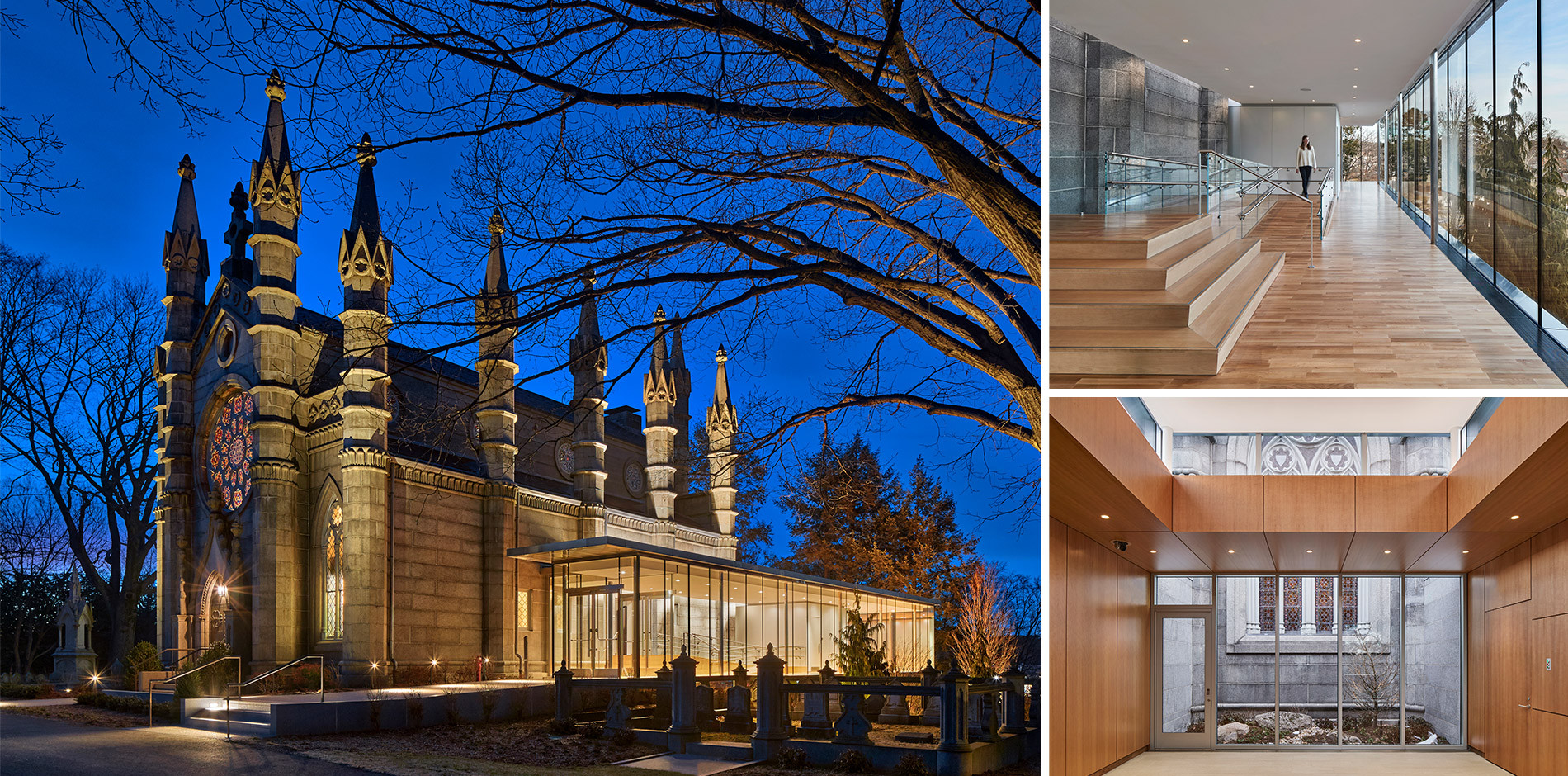This photo collage features three images, with the largest on the left and two smaller ones on the right. The prominent left photo, taken just after dusk against a dark blue sky, depicts an old, castle-like church illuminated by fog lights. This church boasts a large round stained glass window at the front, several spires, and columns along its sides. Adjacent to the church is a modern glass addition, separating it from an adjacent graveyard. The glass enclosure, bright with interior lighting, reveals wood floors and a staircase inside. The top right image affords an internal view of this glass addition, showing a person standing on the wooden floor. The bottom right image further highlights the interior, featuring glass doorways and wooden walls, with the left side retaining the original church façade. Together, these photos illustrate the blend of historical architecture with contemporary renovation.